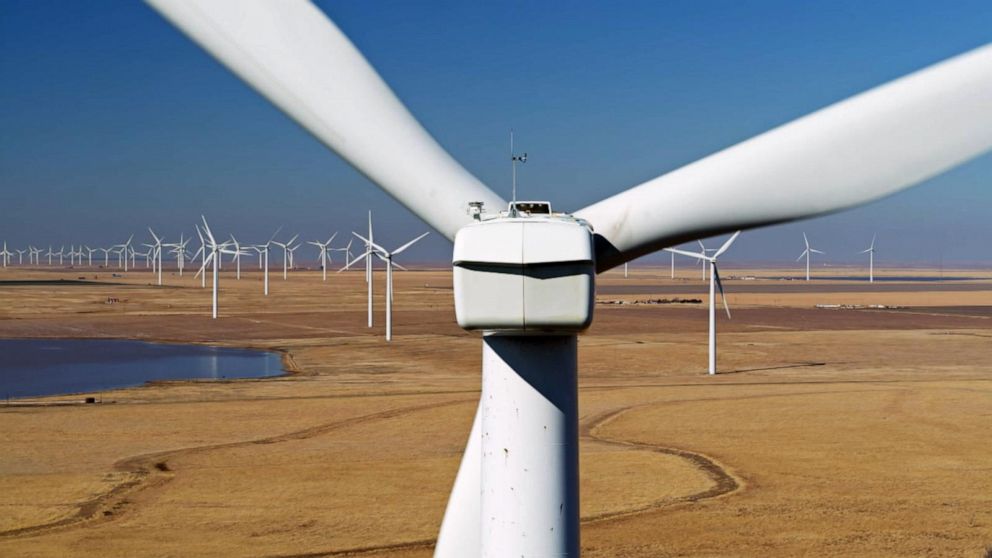This image captures a vast wind farm in a dry, barren landscape, dominated by rows and columns of white wind turbines that stretch into the distance. The foreground is framed by the massive blades and central hub of a large turbine, providing a sense of scale to the towering structures. The landscape below is characterized by a tan to brown soil, interspersed with patches of dry vegetation and a few small paths, indicating infrequent vehicular or water activity. To the left, a small pond reflects the clear, vivid blue, cloudless sky above. The almost desert-like terrain reinforces the harsh dryness of the area. The central turbine exhibits a detailed view of its housing, with visible scientific equipment and what appears to be an antenna. This wind farm, a testament to renewable energy, is set against a backdrop where the natural and mechanical elements sharply contrast yet harmoniously coexist.